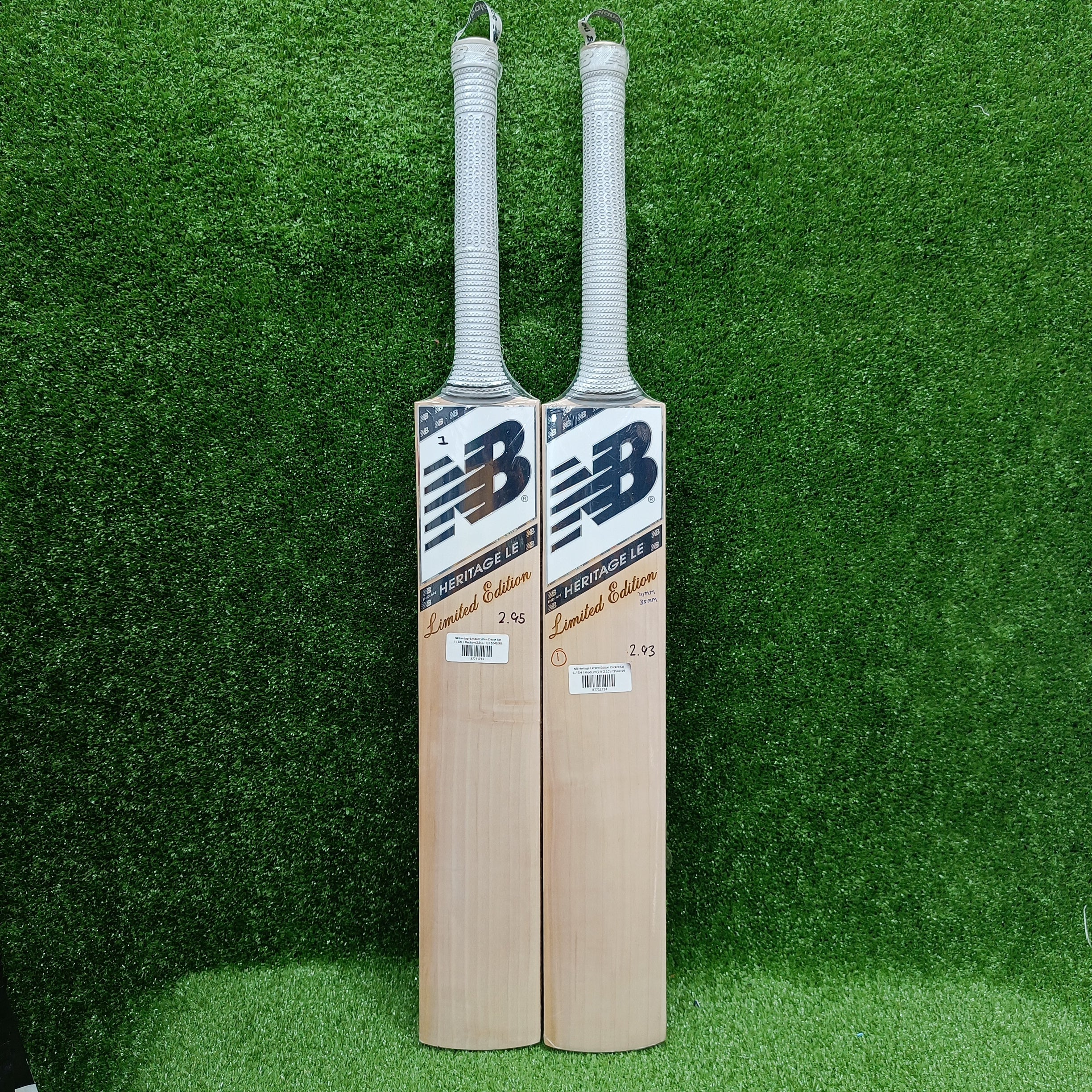The image features two cricket bats positioned side-by-side, leaning against a wall covered in artificial green turf. Both bats have gray handles that appear to be wrapped in a textured fabric or plastic, and are made of light-colored wood. The bats are long and flat, resembling fan blades. Prominent on the bats are the markings "NB", "Heritage LE Limited Edition", and the numbers "2.95" and "2.93". Each bat also has a barcode label affixed to it. The entire scene is set against a backdrop of fake grass, giving a sporty yet synthetic ambiance.